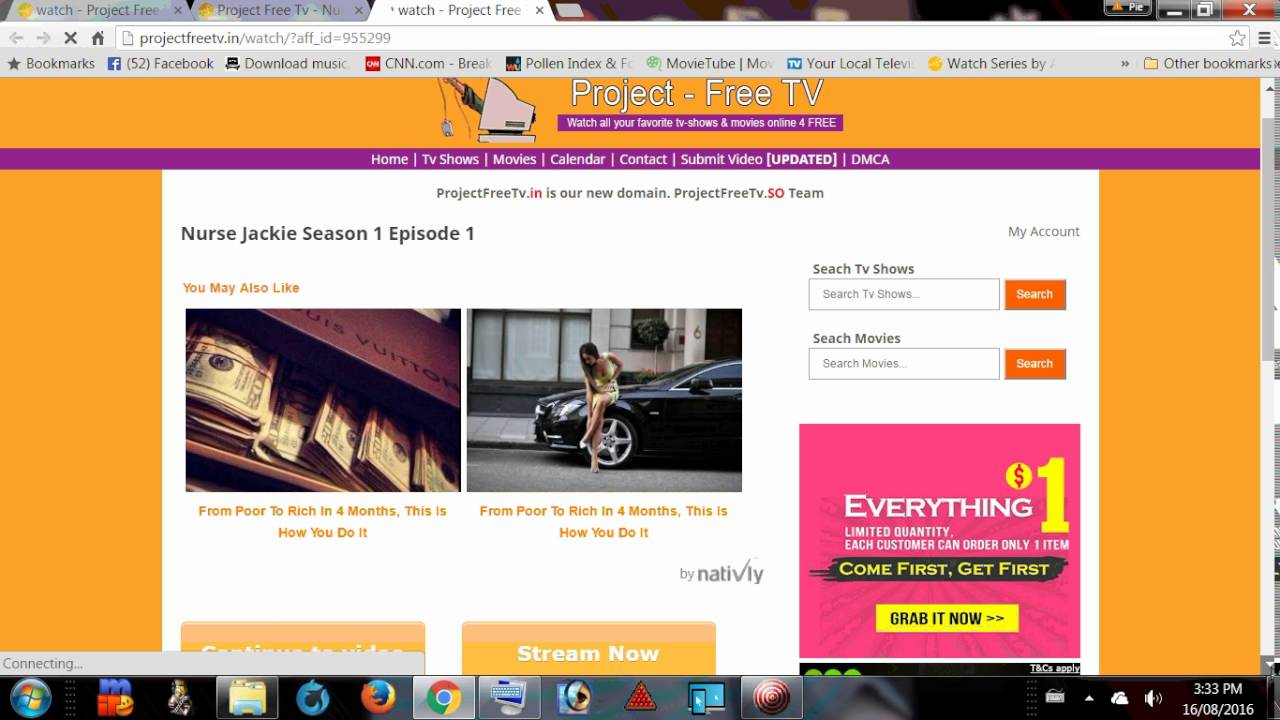The image is a screenshot of a video streaming website called "Project Free TV." At the top center of the webpage, the platform's name, "Project Free TV," is prominently displayed, accompanied by the tagline, "Watch all your favorite TV shows and movies online for free." Just below this, in the left section of the image, there is a listing for "Nurse Jackie Season 1 Episode 1." Alongside this listing are two repetitive promotional links titled, "From Poor to Rich in Four Months: This is How You Do It." Above these promotional links are images, including a briefcase filled with money and a woman standing against a car, presumably to entice viewers with the promise of quick riches.